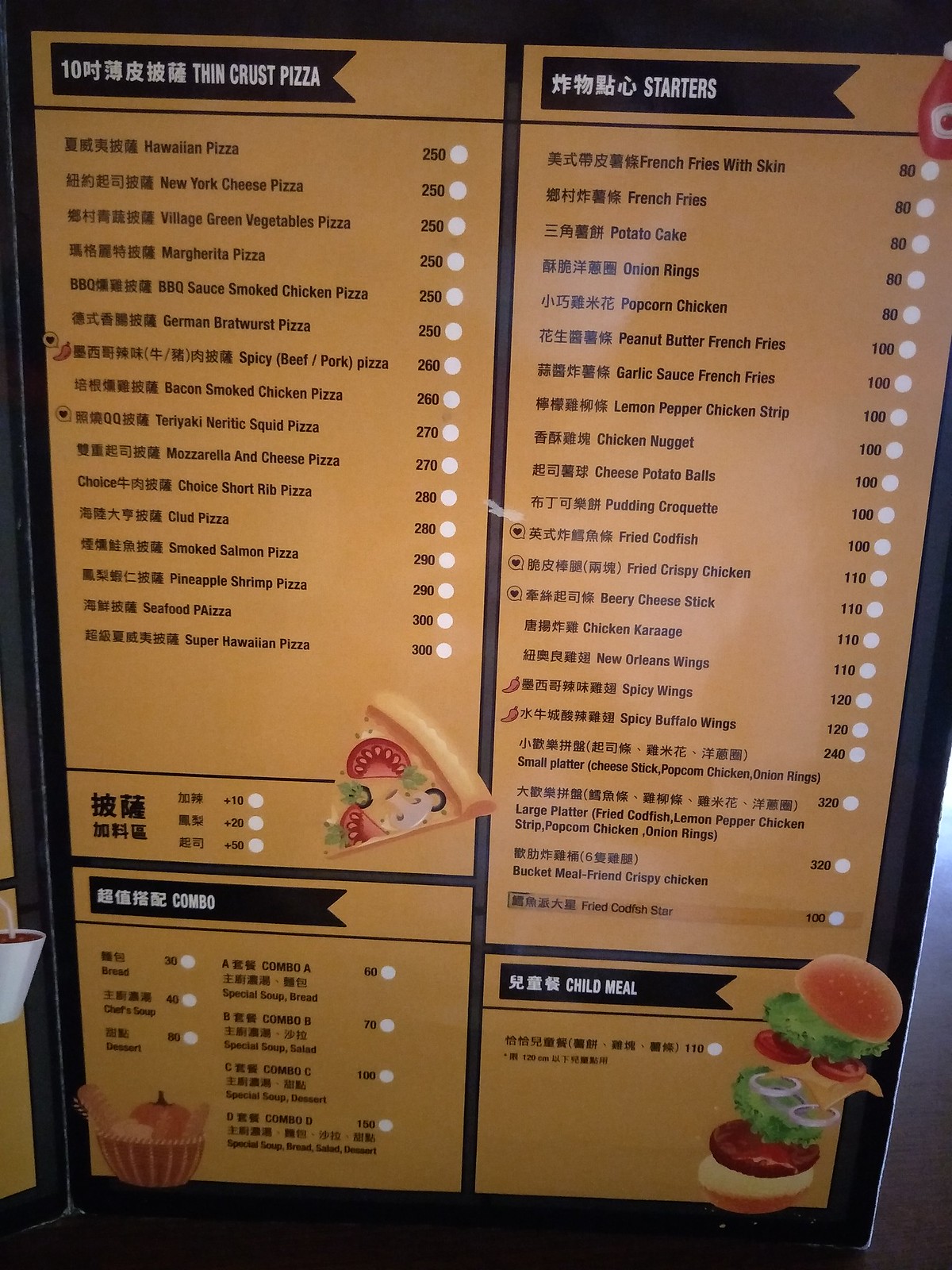The image features a menu set against a neutral gray background. The menu is open, displaying the right page prominently. The layout is predominantly in Chinese with occasional English translations. At the top part of the menu, there are two black ribbon banners. The left banner reads "Thin Crust Pizza," while the right one says "Starters." The main background of the menu is a warm brown color.

On the left side of the menu, Chinese text is listed with English translations and corresponding prices next to each item. The section also includes a small graphic of a pizza slice at the bottom right side. Below this section, another black ribbon banner marked "Combo" appears, accompanied by Chinese text and an image that resembles a basket with a pumpkin in it.

The right side of the menu underneath the "Starters" section includes Chinese characters alongside listed English food items and their prices. Beneath this, there is another black ribbon banner labeled "Child Meal," featuring a deconstructed cheeseburger with all its toppings artfully suspended in the air above it.